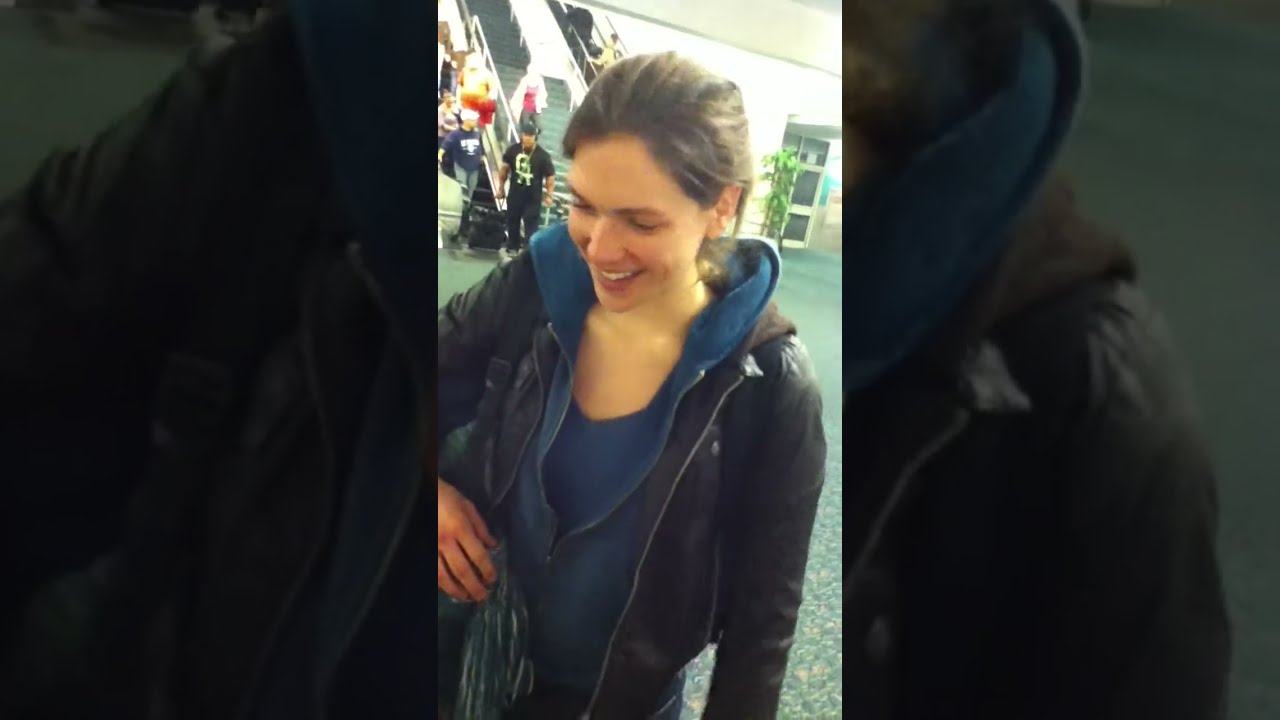The photograph, taken indoors at a busy shopping mall, is framed with a thick black border on the left and right sides, making only the center third visible. This vertical shot captures a scene bustling with activity. Central to the image are two pairs of downward-moving escalators, situated right next to a staircase. Most people are riding the escalators, which are filled with shoppers, while only a few are seen descending the staircase. The ceiling overhead features a gray grid design with a light in the upper right-hand corner, and the floor below is a grayish color, possibly carpeting. Alongside the escalators and stairs, groups of people are visible, including a woman carrying shopping bags and others with purses. In the background, there are more people, some heading towards the left side of the image. A few men and women can be spotted amid the crowd. Additionally, there is a plant placed in one of the corners, adding a hint of greenery to the scene.